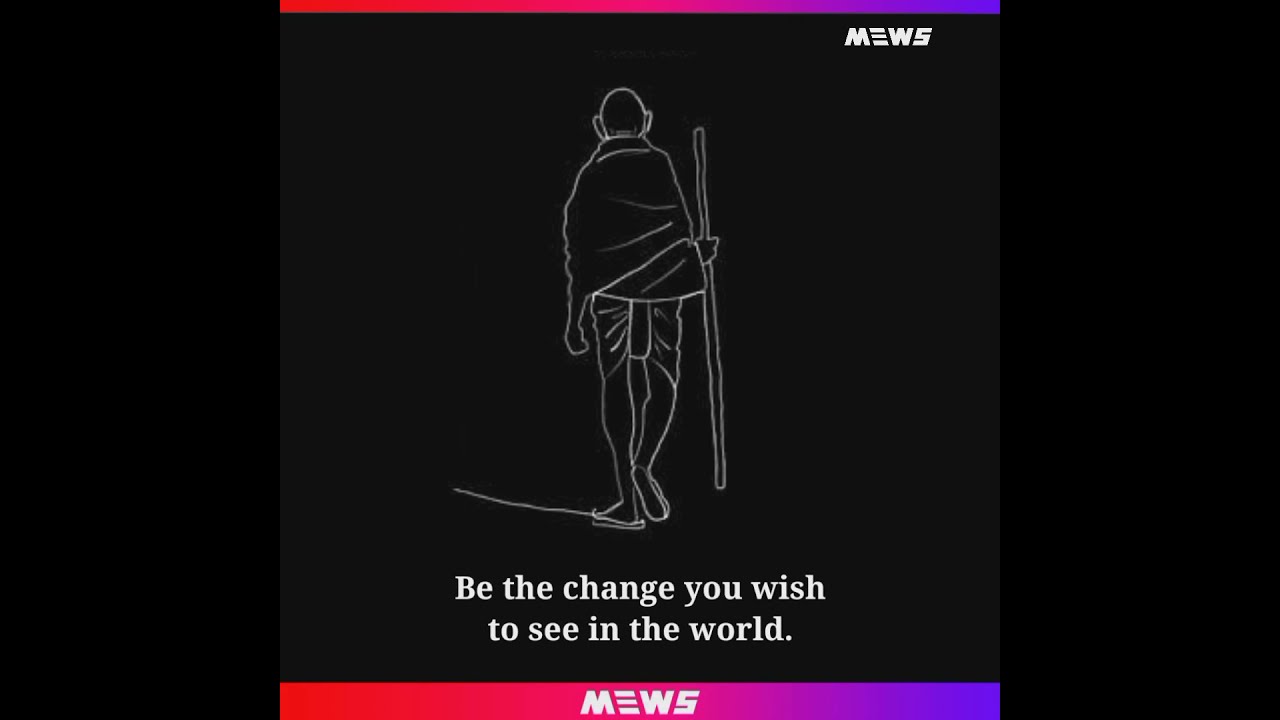The image is a line drawing with a black background and white line work, depicting a figure walking away while holding a walking stick in their right hand. The figure, possibly representing Gandhi, is draped in what appears to be a toga or wrap, with sandals visible on their feet. The background is predominantly black, with lighter and darker shades differentiating the areas. Flanking both sides of the drawing are wide, very dark black vertical bars. 

Above the figure’s left foot is a line extending outwards, suggesting a path. At the upper right corner of the image, there is text reading "M-E-W-S," which also appears at the bottom within a red and purple gradient bar. The top of the image features a thinner bar with the same gradient. Beneath the drawing is a meaningful quote in white text: "Be the change you wish to see in the world." The lettering of "M-E-W-S" at the top forms a unique font, where the "E" is stylized with three lines stacked on each other.